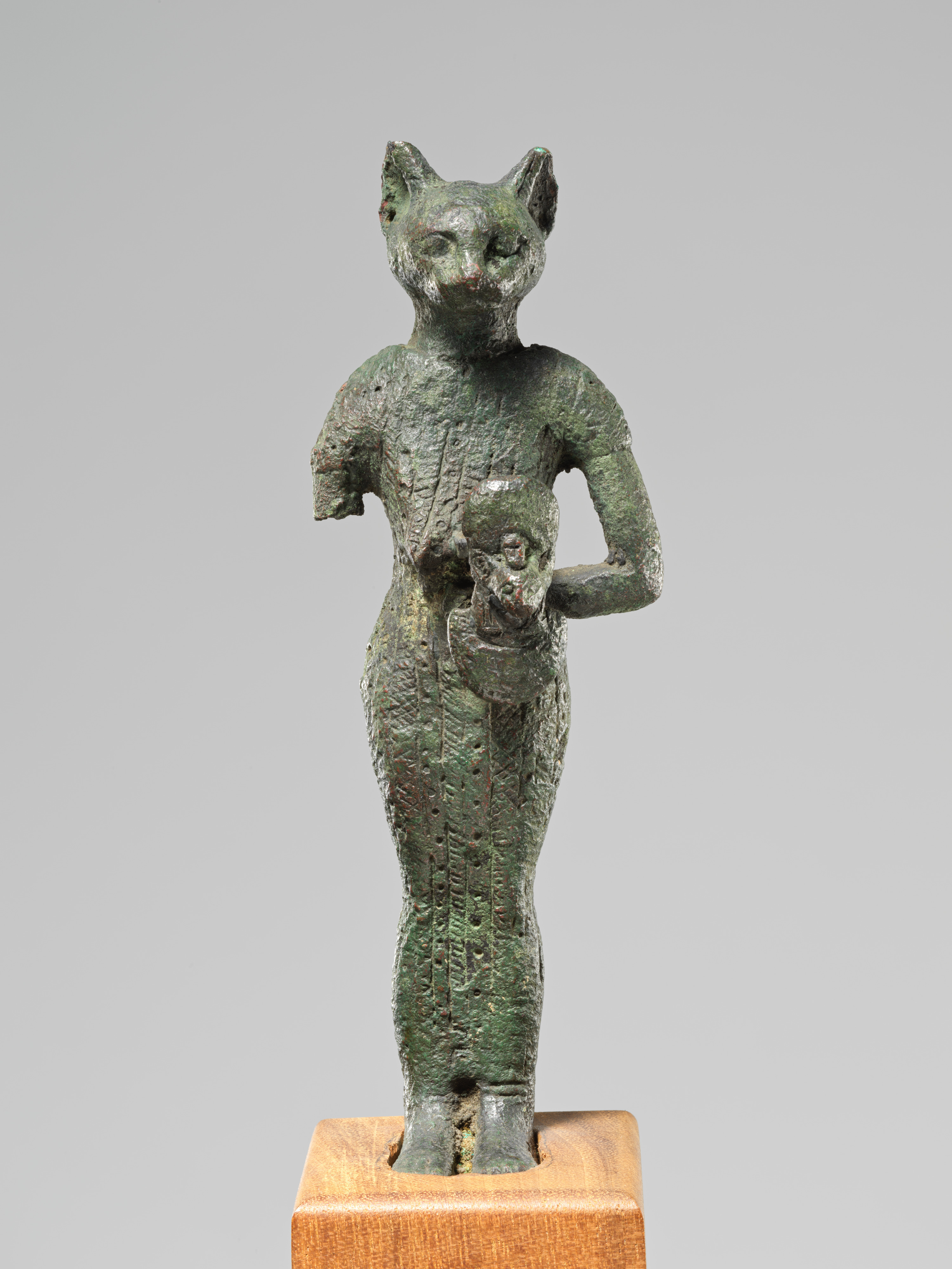This photograph showcases a faded bronze statue of an Egyptian cat deity, depicting a bipedal figure with a cat's head. The statue, weathered and green from verdigris, stands on a beige or orange-ish wooden pedestal. The detailed carvings on its surface, both horizontal and vertical, suggest it is an ancient artifact displayed in a museum or gallery. Notably, the statue's right arm is broken off, while its left arm cradles a smaller cat statue, indicating its value. The background is a plain gray, emphasizing the piece's prominence, as one would expect in a curated exhibit.